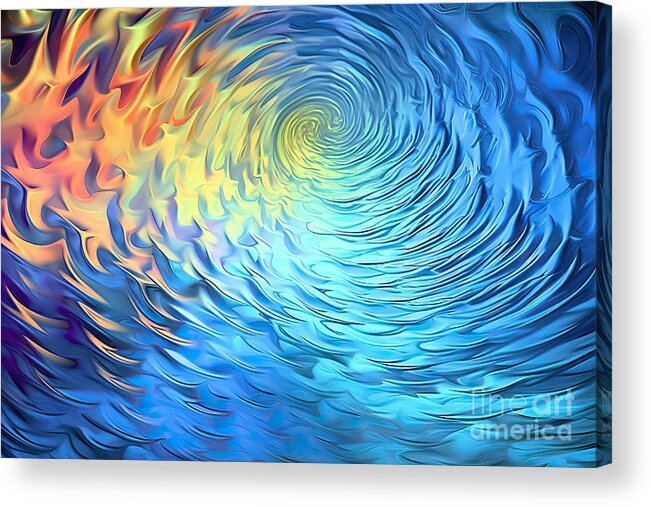This abstract painting evokes a swirling vortex, resembling a whirlpool or a wave, predominantly using shades of blue that transition from lighter hues in the center to darker tones at the edges. The swirling pattern, moving in a clockwise circular motion, is infused with accents of yellow, orange, and a yellowish-orange, creating a vibrant and dynamic contrast. The center of the vortex is situated slightly above the midpoint of the canvas, radiating with a bright burst of color that gradually deepens as it spirals outward. The overall effect is reminiscent of Van Gogh's "Starry Night," capturing a similar sense of movement and color interplay. In the bottom right corner, in translucent white lettering, it reads "Fine Art America," signaling the piece's affiliation. The image contains no figures, structures, or machinery, allowing the viewer's focus to remain solely on the mesmerizing swirl of colors and the fluidity of the composition.